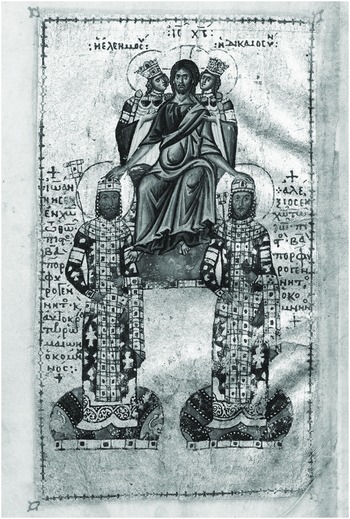The image appears to be an ancient and weathered religious scroll featuring a detailed black and white drawing. At the center of the image, a robed figure, possibly Jesus, is depicted seated on a throne. This central figure is flanked by two kings, identifiable by their crowns and royal garb, who appear to be leaning in to kiss him on the cheeks. Beneath the throne, two tall guards with peculiar checkered patterns on their clothing stand with the seated figure's hands resting atop their heads. The border of the scroll is adorned with numerous small crosses, adding to the religious motif. Despite the presence of some written text, its language remains indeterminate, blending with the overall black and white aesthetic of the artwork.